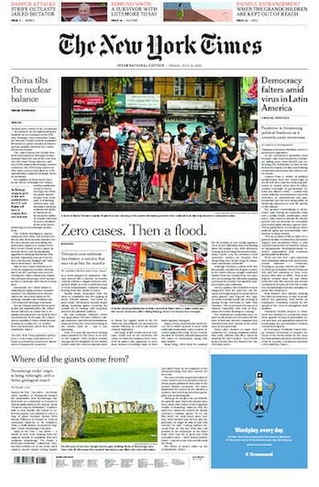The screenshot captures a web page resembling the New York Times website. At the top center of the page is the iconic New York Times logo, immediately grounding the viewer in the context of the publication. Just below the logo, there is a prominent photograph showing a group of people standing together, seemingly on a street, possibly participating in a public gathering or event.

To the left of this central image is a headline that reads, "China Tilts the Nuclear Balance," suggesting a story about geopolitical shifts related to nuclear capabilities. On the right side of the image, another headline declares, "Democracy Falters Amid Virus in Latin America," indicating an article focused on the political and social impacts of a health crisis in that region. Below these main features, a smaller headline reads, "Zero Cases, Then a Flood," hinting at a dramatic development following an initial period of stability, presumably related to virus cases.

This detailed web page representation captures a moment in time, reflecting critical global issues spanning political power dynamics, health crises, and their far-reaching consequences.